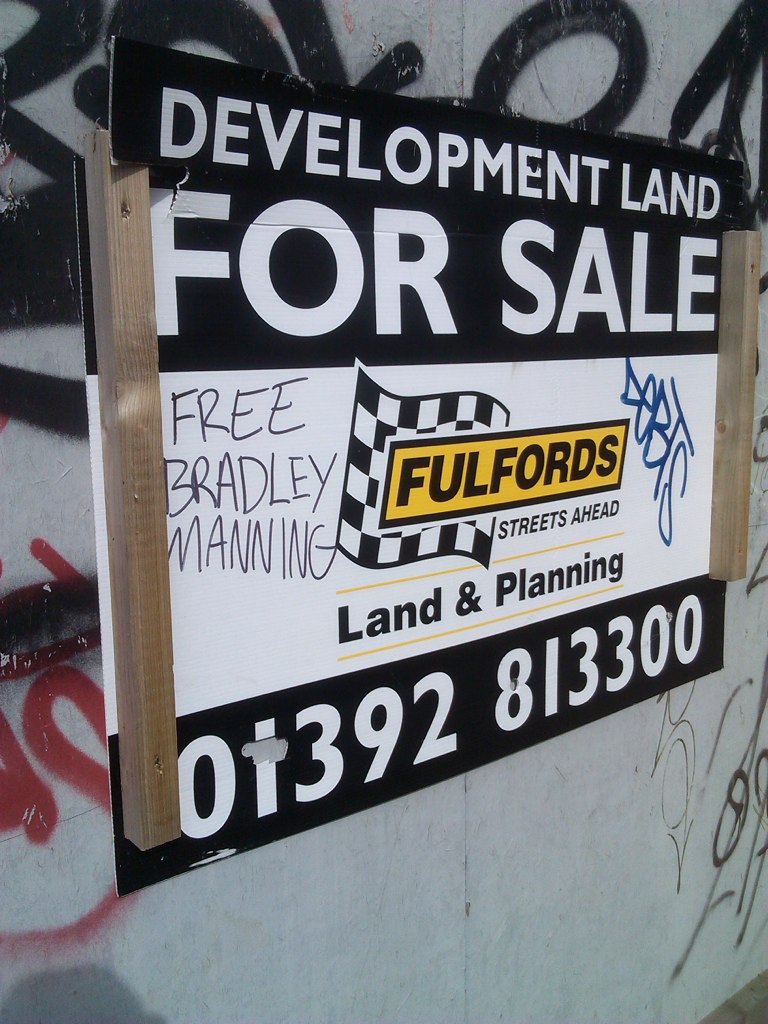This image showcases a sign attached to a wall, bordered by wood, and partially defaced with blue graffiti on the right side. At the top, the sign features a black background with bold white letters stating, "Development Land for Sale." Beneath this, the main portion of the sign has a white background, interrupted by a checkered flag graphic with black and white squares. Centrally located on this white section is a yellow box inscribed with black letters reading "Fulfords." Below this, also on the white background, it states "Streets Ahead," followed by a thin yellow line. Underneath this line, it says "Land and Planning," followed by another yellow line. At the bottom, the sign returns to a black background with bold white letters showing the phone number "01392-813300." Additionally, the phrase "Free Bradley Manning" is visible, scrawled by hand across the sign.